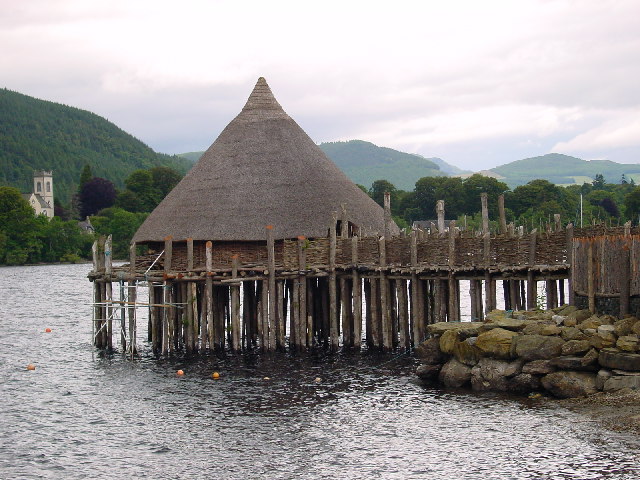The photograph captures an outdoor scene, taken during the daytime under an overcast sky. The setting centers around a large body of water, either a lake or a river, which appears dark in color, reflecting the subdued lighting of the day. In the foreground, at the lower right, a pile of rocks meets the brown dirt of the shore. A wooden deck with a natural wooden wall, constructed from sticks or logs, extends towards a distinctive round, thatched building. This structure, reminiscent of traditional rice paddy hats, features a cone-shaped roof and walls made of thatched materials, standing on a dock supported by sturdy cut timber logs elevated above the waterline.

To the left, a prominent building resembling a church with a bell tower is visible, providing a focal point in the midst of lush, green hills and small mountains that fill the distant background. These hills, densely covered in verdant foliage, contribute to the serene and somewhat native atmosphere of the scene. The entire backdrop is a canvas of deep green trees under a cloudy, white sky, enhancing the overall sense of calm and natural beauty in the photograph.